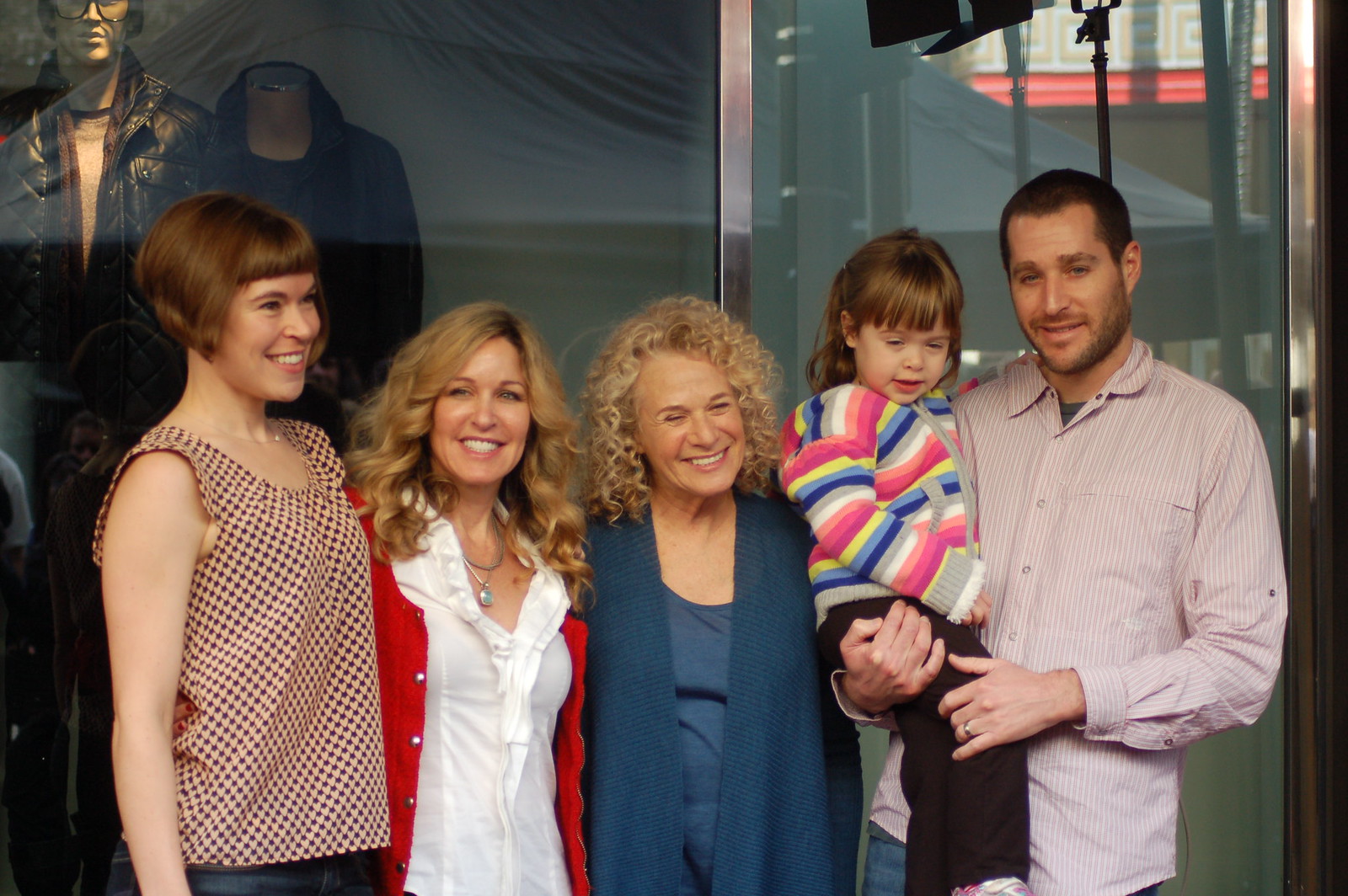In the photograph, a family is posing in front of a clothing store, all smiling broadly. On the right side, a man with short brown hair is holding a young girl in his right arm. The man is dressed in a light-colored, striped button-down shirt, while the little girl wears a striped hoodie and black pants, showcasing her medium-length brown hair. Centrally positioned is a middle-aged woman with curly blonde hair, donning a blue sweater over a blue undershirt. To her left, a blonde woman with an open white shirt and a red sweater stands, her long blonde hair framing a cheerful smile. On the far left, another woman with a short, hazel bob haircut is clad in a patterned, sleeveless checkered shirt, also smiling. Behind her, a mannequin dressed in a black leather jacket and sunglasses subtly adds to the scene.